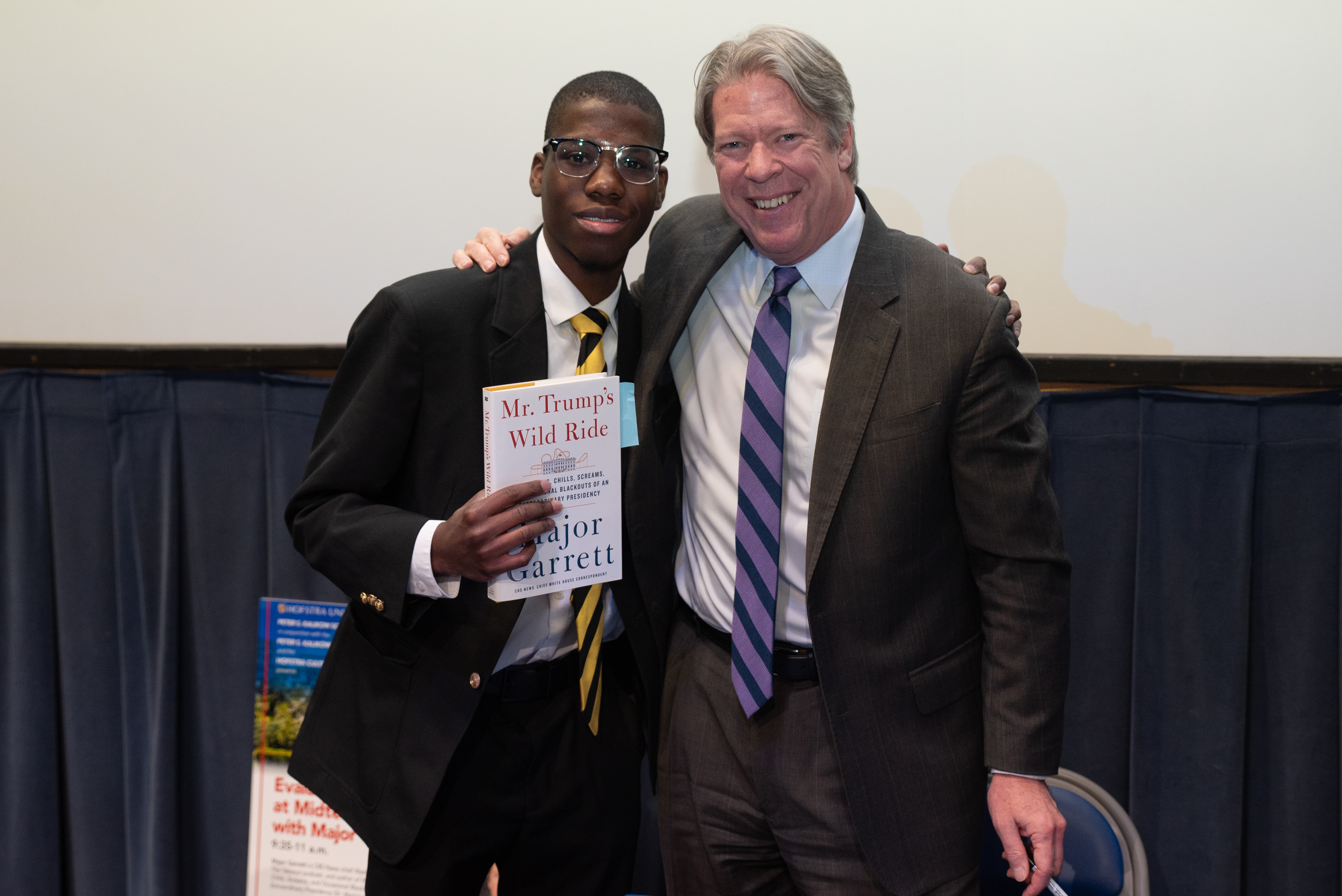In the image, Chief Washington Correspondent for CBS News, Major Garrett, and a young man stand arm in arm, both dressed in suits, ties, and white shirts. The young man holds a copy of Major Garrett’s book, "Mr. Trump's Wild Ride". The setting suggests a book release event or convention. Behind them, there is a poster on the floor near the man on the left, partially obscured by a backdrop with beige and grape-colored sections. To the right, there's a folding chair and curtains adding to the ambiance. The scene is brought to life with a variety of colors including yellow, black, dark blue, light purple, tan, brown, blue, light blue, red, and greens.